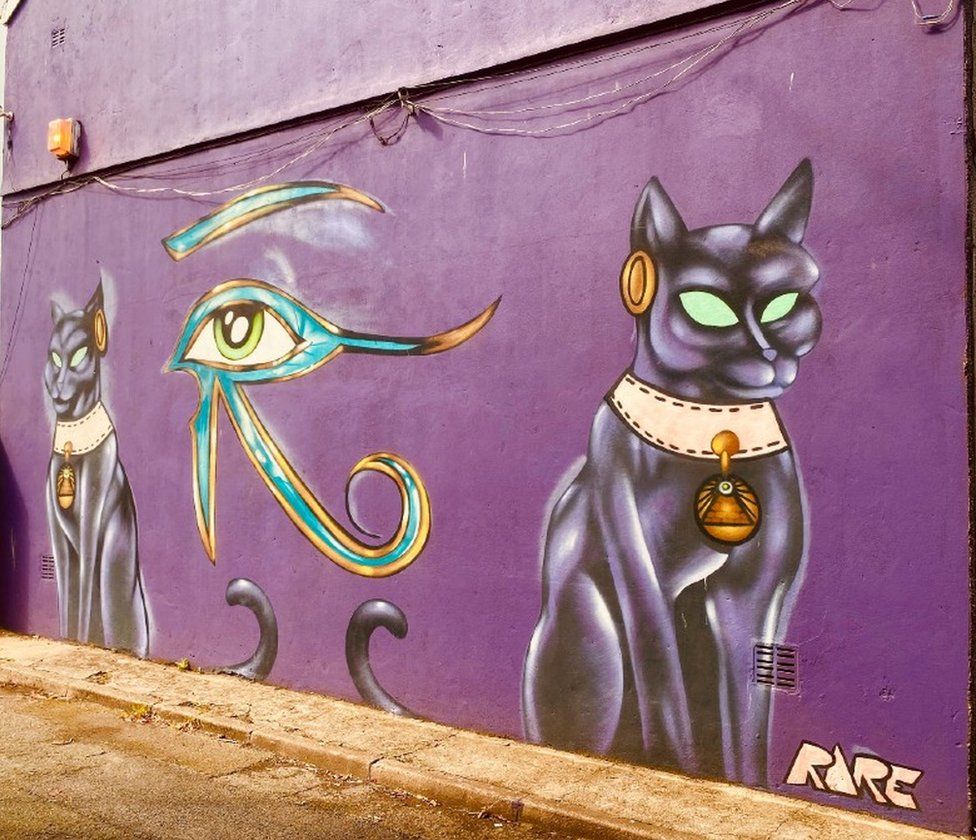The image features a vibrant graffiti mural painted on the side of a building with a striking purple background. Dominating the mural are two sleek, black, robotic-looking cats with piercing green eyes devoid of irises. These cats are adorned with white collars and golden pyramid pendants. One cat is located on the far right side of the mural, while the other is positioned to the left. Centrally placed between the cats is an intricate depiction of the Eye of Ra, featuring a turquoise outline and a green iris with a black pupil. The word “RARE” is inscribed in white text at the bottom right corner of the mural. The setting includes a light brown walkway, possibly made of bricks or cement, and an asphalt road. Adding to the scene's urban character are visible electrical wires and an orange light fixture on the wall, enhancing the ancient Egyptian theme of the graffiti.